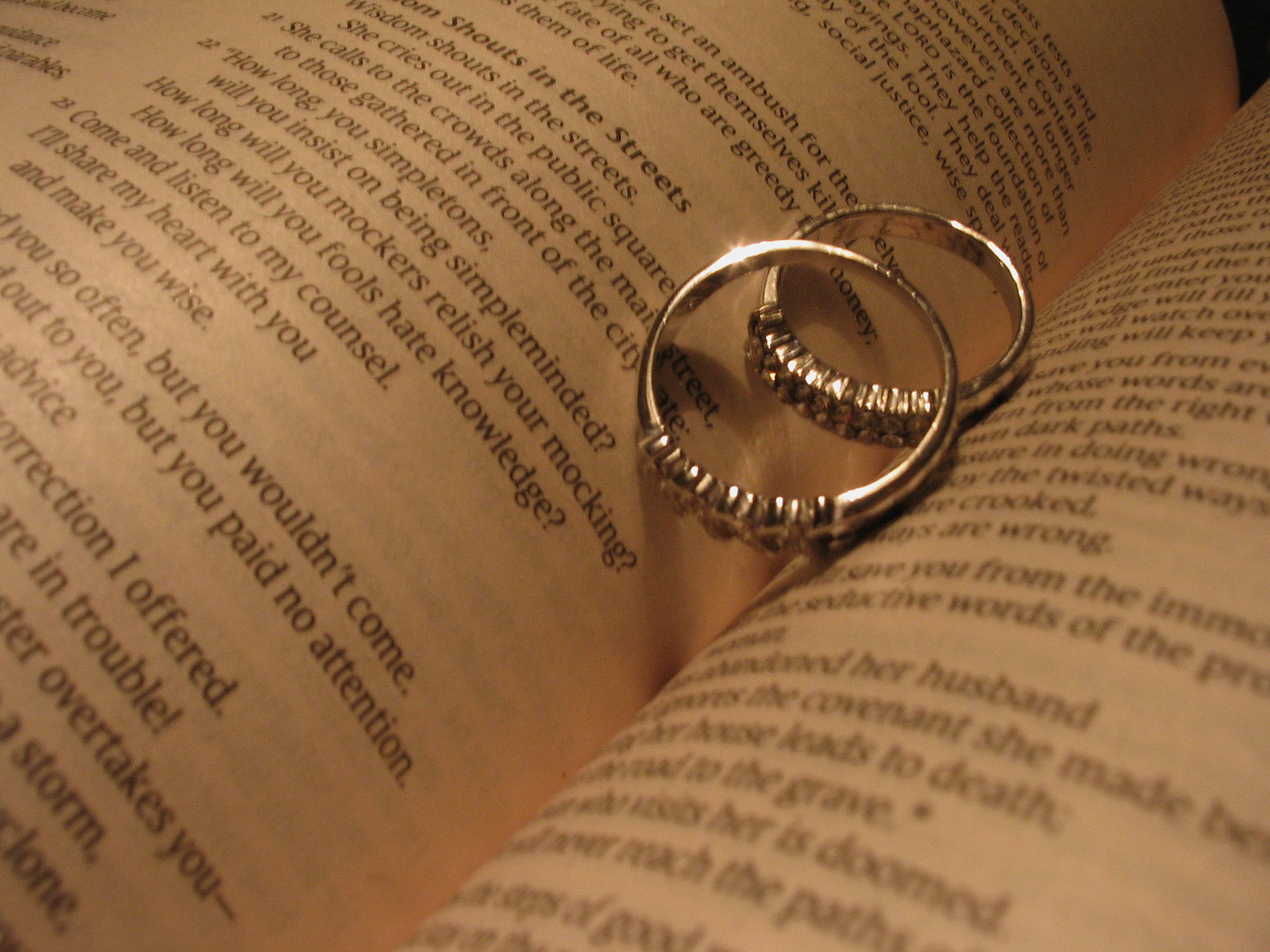The image depicts a close-up of an open book with white pages and black text, positioned indoors, possibly in a bedroom or library. The book, appearing to feature poetry or Biblical text, serves as the background. In the foreground and central to the image are two overlapping wedding rings nestled in the valley where the pages meet the spine. These metallic rings, adorned with gemstone fixtures on one side, create a striking focus against the textured expanse of text. The minimal black background provides contrast, ensuring that the rings and book are the primary elements in this serene and intimate composition.